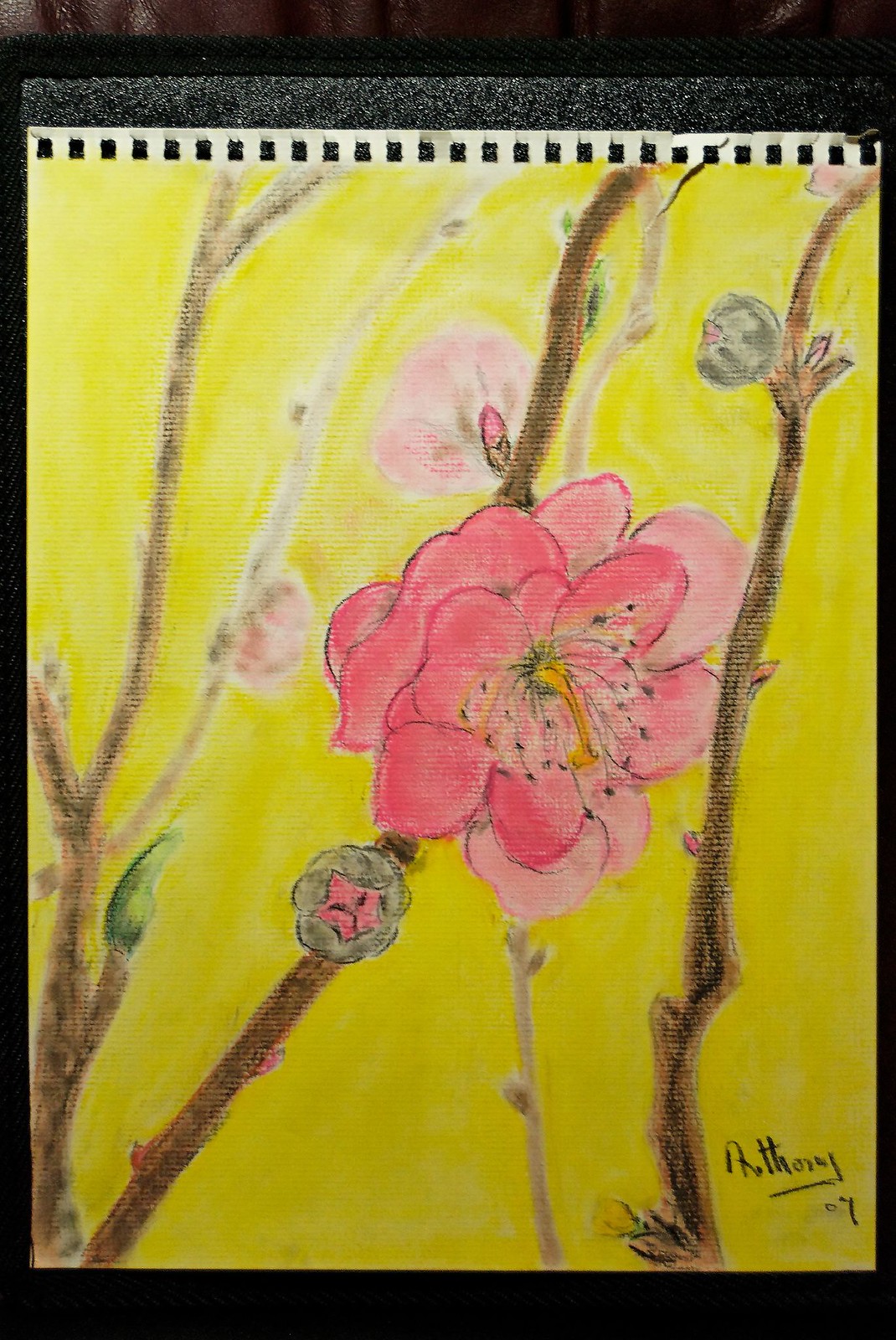A delicate and detailed sketch seems to have been torn from a notebook or sketchbook, as evidenced by the visible coil marks at the top edge of the paper. The background is a vibrant, almost luminous yellow, providing a striking backdrop to the intricate drawing that overlays it. In the center, a large, exquisitely detailed pink flower draws the viewer's attention, featuring petals in varying shades of dark and light pink that give it a sense of depth and texture. Surrounding this focal bloom are brown branches bedecked with smaller buds and faintly sketched flowers, lending a realistic botanical touch. The entire composition has a dreamy, ephemeral quality, with some flowers appearing softer and less defined, creating a sense of depth. In the bottom right-hand corner, the artist's name, "Anthony," is subtly etched, along with a possible date, which reads either '04 or '09. This touch adds a personal and historical element to the artwork, inviting viewers to ponder the story behind it.